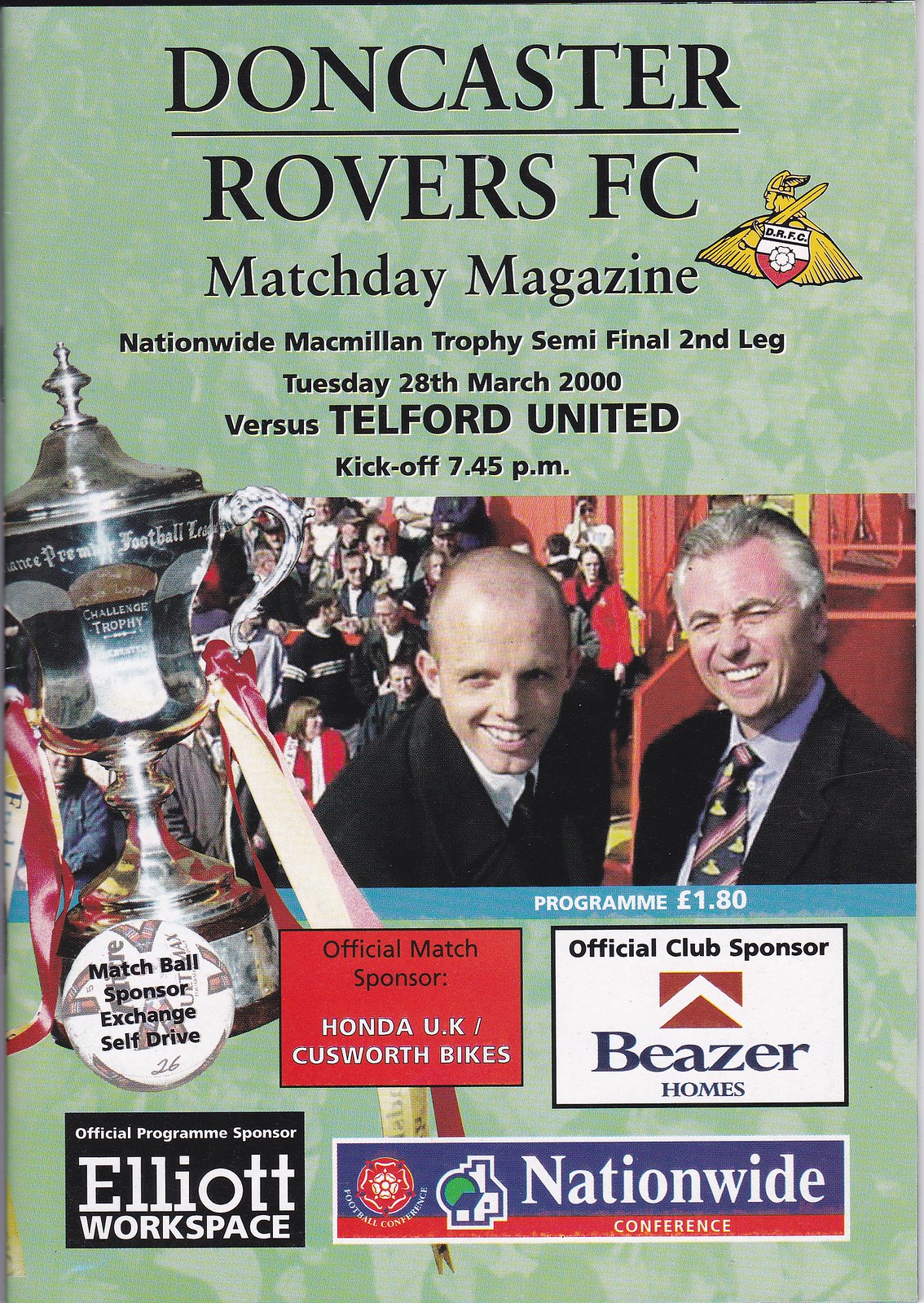The image depicts a magazine cover primarily featuring Doncaster Rovers FC. The background is a blend of light blue-green hues with white patches. Dominating the top portion in bold black, all-capital letters, is "DONCASTER," and below it reads "ROVERS FC." The header includes a logo showcasing a yellow emblem of a man with a sword and shield, the shield being white and red.

In elegant black text beneath the header, it states "Match Day Magazine", followed by details of the event: "Nationwide Macmillan Trophy Semi-Final Second Leg." The specific date and matchup are clearly listed: "Tuesday 28th March 2000 vs Telford United," with the kickoff time set for 7.45 pm. 

On the left side, there is a silver and gold trophy labeled "Matchball Sponsor Exchange Self-Drive." Further details on this cover highlight event sponsors such as "Official Match Sponsor Honda UK / Cusworth Bikes," with a red background, and "Official Club Sponsor Beezer Homes," featuring a logo that includes a "V," situated in a white box. Additionally, the "Official Program Sponsor Elliott Workspace" is backed by a black square, while a nearby "Nationwide Conference" logo is placed within a red, white, and blue rectangle.

Also prominently featured is a picture of an enthusiastic crowd at a stadium and two men in suits; the older man, who is bald and smiling, wears a dark suit, while the other, also smiling, has gray hair and sports a pink, navy, and yellow striped tie. They both stand out against the backdrop, which includes more spectators.

Overall, the colors present in the image include red, white, silver, gold, blue, green, gray, yellow, and black, adding a vibrant touch to the cover. The cover price is marked as £1.80.